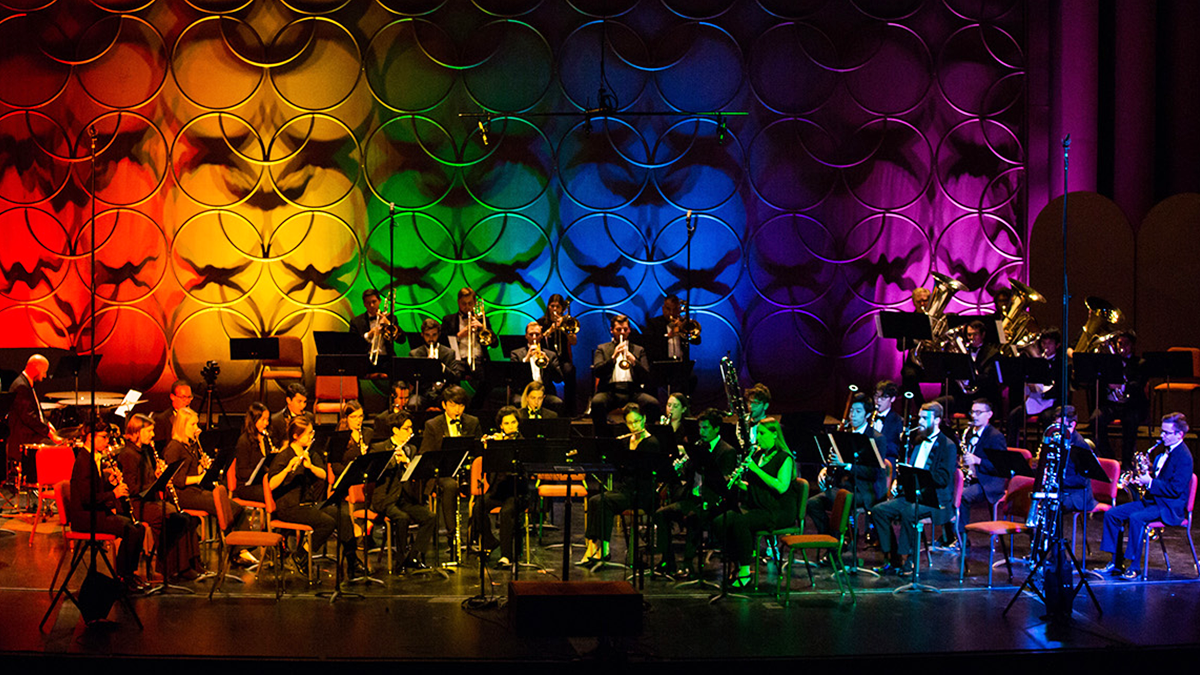In this vibrant photograph, an orchestra is seated on a stage, immersed in the hues of rainbow-colored lights projected from above. The stunning lighting, transitioning seamlessly from orange to pink with distinct sections of red, yellow, green, blue, and purple, creates a vivid backdrop. These colors wash over the musicians, casting them in corresponding shades and adding a dynamic visual element to the performance.

The orchestra is arranged with wind instruments prominently featured. To the left are flutists, while the right side reveals trombones, trumpets, and even large brass instruments such as tubas positioned in the back. Woodwind instruments like saxophones and clarinets are scattered among the musicians, who are formally dressed in tuxedos and elegant black attire. Additionally, there's a pianist on the far left and a percussionist seated behind a drum set further to the left.

Large circular metal rings adorn the wall behind the orchestra, adding depth and enhancing the thematic presentation, hinting at a possible celebration of diversity, as suggested by the pride flag colors. This richly detailed scene combines musical artistry with a powerful, colorful display, capturing the essence of a symphony performance with a modern, inclusive twist.